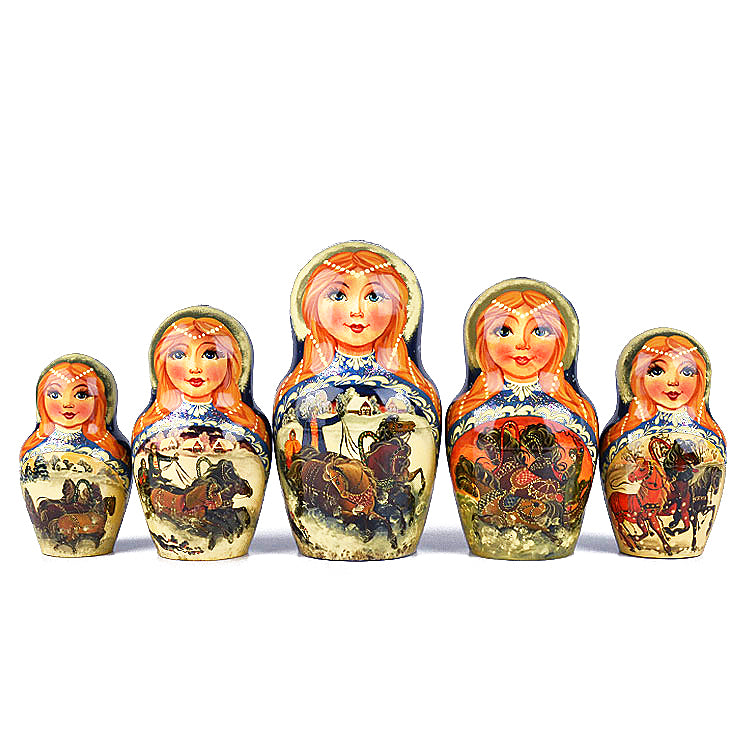This image showcases a set of five traditional Russian Matryoshka dolls, each progressively smaller and nestled within the next. At the centerpiece stands the tallest doll, flanked symmetrically by four smaller dolls on either side. The figures are intricately painted to depict a young redheaded woman adorned with a beaded pearl wreath that drapes over her shoulders. Each figurine has striking blue eyes and wears a blue, lace-bordered collar with various patterns.

The lower halves of these dolls vividly illustrate a picturesque snowy day, featuring scenes of horse-drawn carriages—a man driving the sleigh in the forefront of the largest doll, with houses and trees painting the backdrop. These scenes appear to narrate a journey, suggesting that the sequence of dolls—from largest to smallest—represents different moments or stages of a story. Dominant colors include shades of orange, white, and blue, adding to the seasonal, wintry aesthetic of the artwork. The overall image is set against a white background, emphasizing the detailed and vibrant craftsmanship of the nesting dolls.